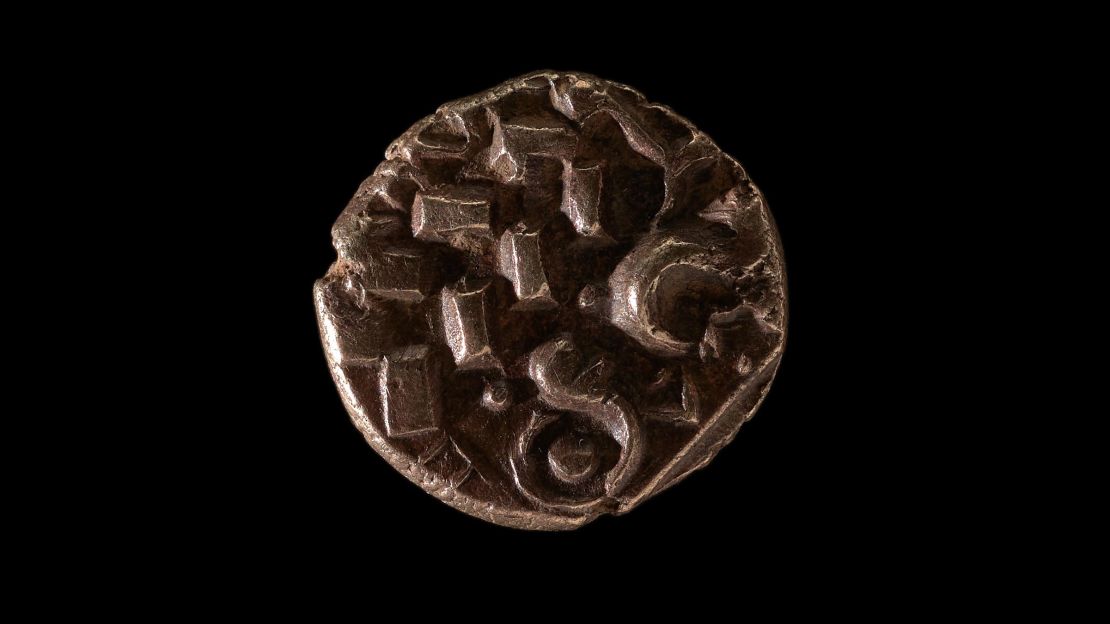The image depicts a small, circular artifact set against a completely black background. The object is dark brown with a slightly uneven, textured surface, suggesting it may be made of metal, stone, wood, or hardened clay. The artifact displays intricate carvings, with prominent rectangular, square, and S-shaped patterns on the top half, and circular and semi-circular shapes on the bottom half. These markings and the worn, imperfect edges hint at its age and possible historical significance. The object appears three-dimensional, with some parts catching the light, giving it varying shades of brown. The details and craftsmanship hint at its potential use as an ancient coin or tool, though its exact purpose remains unclear.